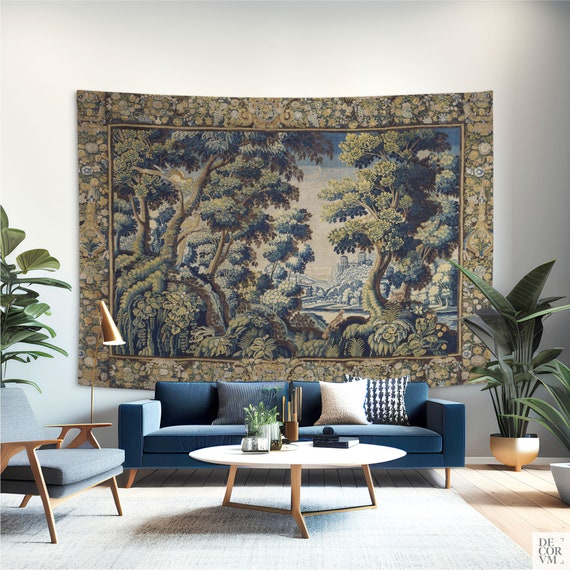This image captures a cozy, well-decorated interior of a home. Dominating the scene is a striking tapestry on a pristine white wall, featuring an intricate design. The tapestry's border showcases green hues interspersed with various flowers, while the central motif depicts a serene woodland scene with detailed trees. Below the tapestry sits a plush blue couch adorned with several soft pillows, flanked by a stylish blue chair with wooden armrests, adding a touch of elegance to the space. 

A large white rug sprawls across the light-colored hardwood floor, providing a cozy contrast and enveloping most of the area depicted in the image. On one side of the couch stands a circular white table, cluttered with various knick-knacks, hinting at the personal touch of the room's inhabitant. Adjacent to the couch, a gleaming gold lamp stands tall, casting a warm glow to the surroundings. Strategically placed potted plants peek from the edges of the frame, adding a sense of freshness and life to the scene. While some elements in the background remain indistinguishable, the overall composition of the room exudes charm and comfort.